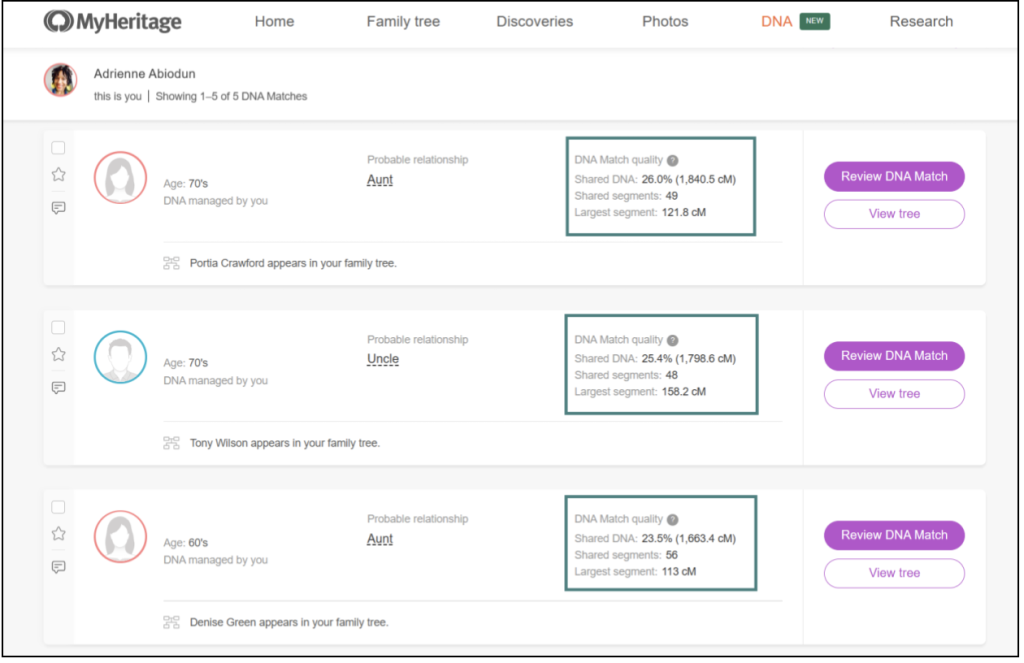This image is a detailed screenshot of the MyHeritage website, an online platform dedicated to exploring ancestry and genealogy. The site enables users to investigate their familial roots, providing extensive insights into their heritage. It also allows users to submit DNA samples for comprehensive ancestral analysis.

The screenshot features a clean design with a white background accented by light gray details. In the top left corner, the MyHeritage logo is prominently displayed, featuring black text with a capitalized "M" and "H" alongside a stylized tree emblem. The top center of the screen contains navigation links labeled Home, Family Tree, Discoveries, and Photos, guiding users to different sections of the website.

Central to the image is a profile belonging to Adrienne Abiodun, who is researching her ancestry. Below her name, three large white boxes are aligned vertically, each offering detailed information about her relatives—two aunts and one uncle. Each box includes the relative's name, age, relationship to Adrienne, and the percentage of shared DNA. On the right side of each box are two prominent buttons: one purple button labeled "Review DNA Match" and one white button labeled "View Tree." These options allow users to delve deeper into DNA matches and explore the family tree connected to each relative.